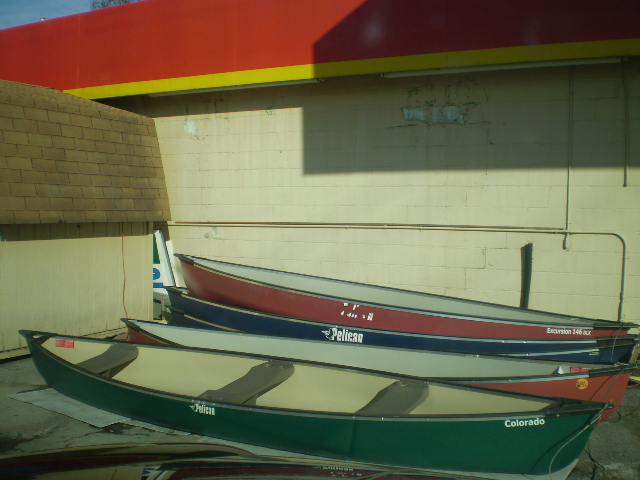The image captures the back of a gas station, featuring a row of canoes aligned horizontally, parallel to each other on a paved surface. These canoes, primarily marked with the "Pelican" logo, display a small mascot of a pelican on the letter 'P'. The prominent canoe in the foreground is green with a beige or light brown interior and equipped with three gray bench seats. This canoe also has the word "Colorado" inscribed on it. Positioned beside it are additional canoes: a red one with a white interior, followed by another red one, then two blue canoes. These canoes are stacked and nested into each other.

The backdrop of the gas station shows a wall made of beige brickwork or stained white cement bricks, exhibiting signs of wear and cracks. A prominent red border with a yellow trim runs across the top of the building. Adjacent to this, on the left side of the image, there is a shed characterized by the same beige coloration on the walls and a darker brown shingle roof. The overall scene has a slightly dilapidated look, indicating a level of neglect.